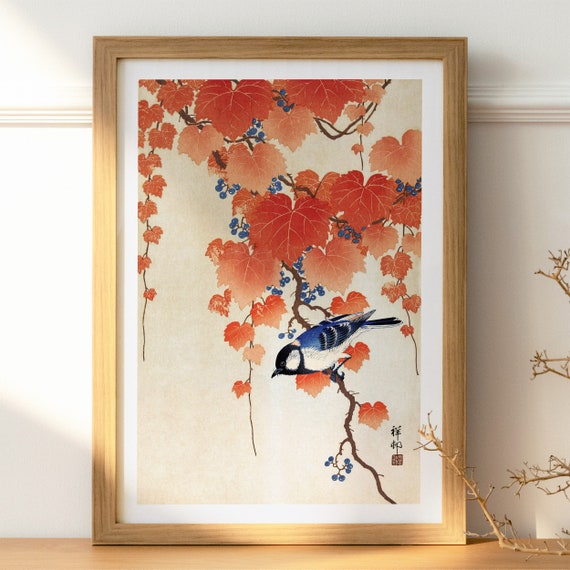The image is a realistic photograph showcasing a framed painting propped up against a white wall with a light wooden floor. The wall features a trim, or molding, roughly one or two feet above the ground. The frame of the painting is a light yellow to medium wood, and it contains a white border around the painting. The artwork depicts a thin, twig-like branch with red leaves varying from salmon to a more pinkish-red hue, and blue berries. A blue and black bird with a white stomach is perched on the branch, approximately two-thirds from the top. The background of the painting is a beige, light stone color. The painting rests on the ground, and in the bottom right corner of the image are visible dried plant stems or branches, adding an organic element to the scene. There is no text within the painting, except for a possible title in Chinese at the lower right corner.